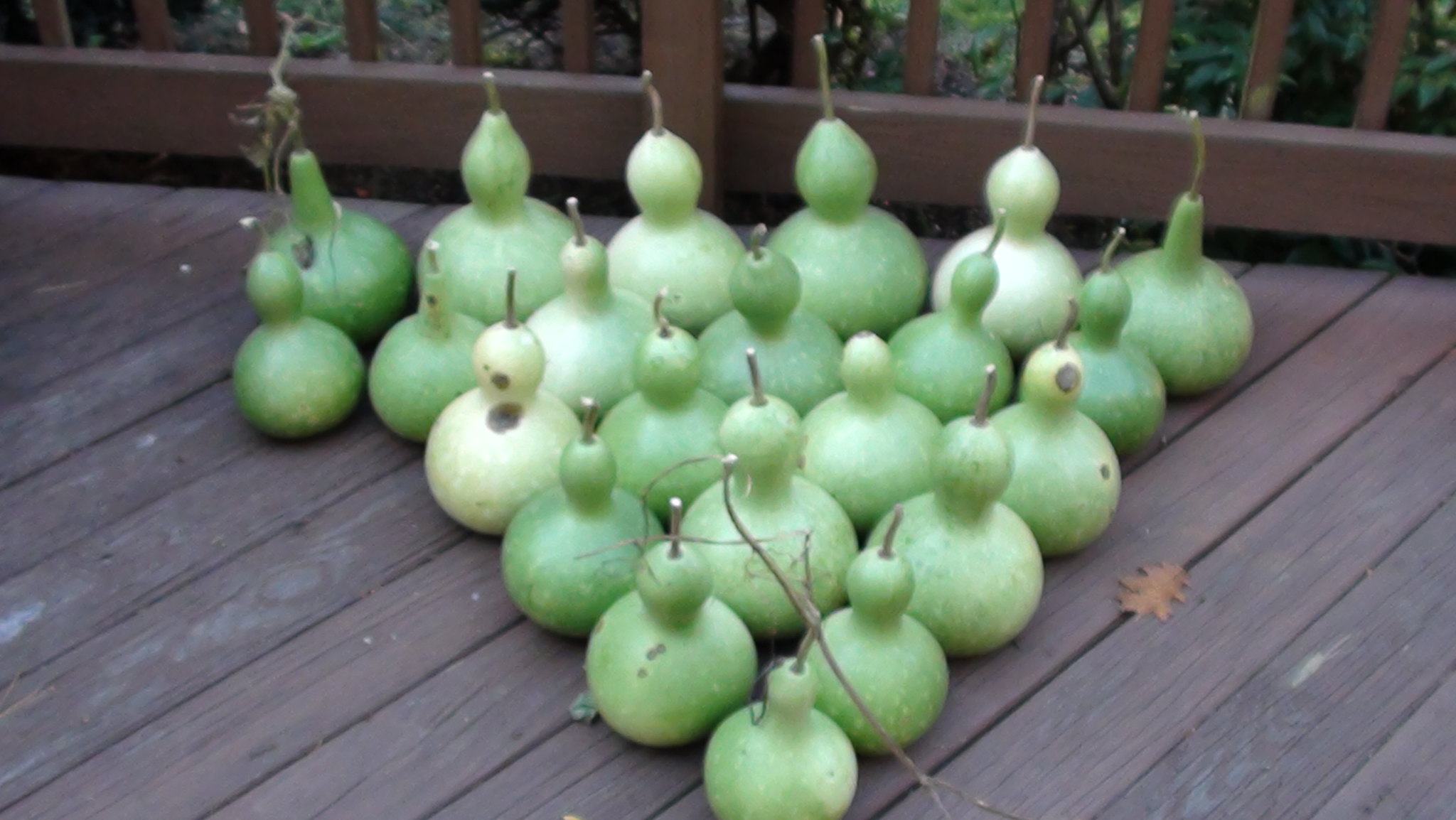The image features a grouping of 22 yellowish-green gourds arranged in a triangular formation akin to bowling pins on a wooden deck. Each gourd, retaining its stem, varies in size from smaller to larger and ranges in color from very pale green to darker green, similar to lime shades. The gourds are bulbous at the bottom with a shorter neck, resembling those used to make birdhouses. The deck, stained a light brown and showing signs of wear with visible scuffs, matches the wooden fence in the background. To the right of the gourds, a single dried leaf can be seen on the deck, adding a touch of natural detail.